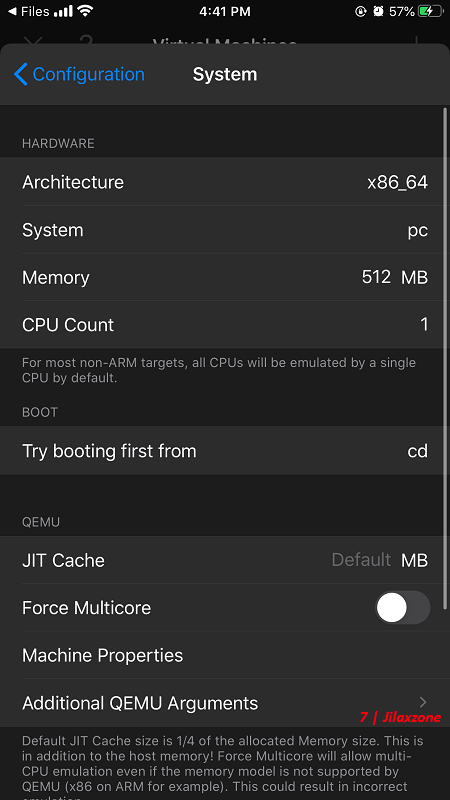The image captures a screenshot taken from a smartphone, presented in a vertical format against a solid black background. The black background lacks any noticeable texture or dimension, giving the screenshot a clean, uncluttered appearance. 

At the top left corner, there is a white arrow pointing left, labeled "Files." Next to it, various status icons display, including a Wi-Fi signal, the word "Sibyl," a signal strength icon, and the time, "4:41 p.m." In the middle section, we see more icons, including a circular arrow, a clock, a battery icon indicating "57%," with the battery status showing that it is charging.

The main focus of the screenshot is on a detailed configuration menu. The first section highlighted is "Configuration," shown in blue text, followed by "System" in white. Below these headers, various categories and pieces of information are listed:

- "Hardware Architecture"
- "System Memory"
- "CPU Count"
- Detailed "Information" section

A specific note mentions, "For most non-ARM targets, all CPUs will be emulated by a single CPU by default."

Continuing down, the menu includes a "Boot" section with configurations such as:
- "Try booting first from a CD"
- "QEMU JIT Cache Default MB"
- "Force Multi-Core" toggle
- "Machine Properties"
- "Additional QEMU Arguments" 

At the bottom, a brief explanatory blurb provides more context, although the content of the blurb is not fully visible in the screenshot.